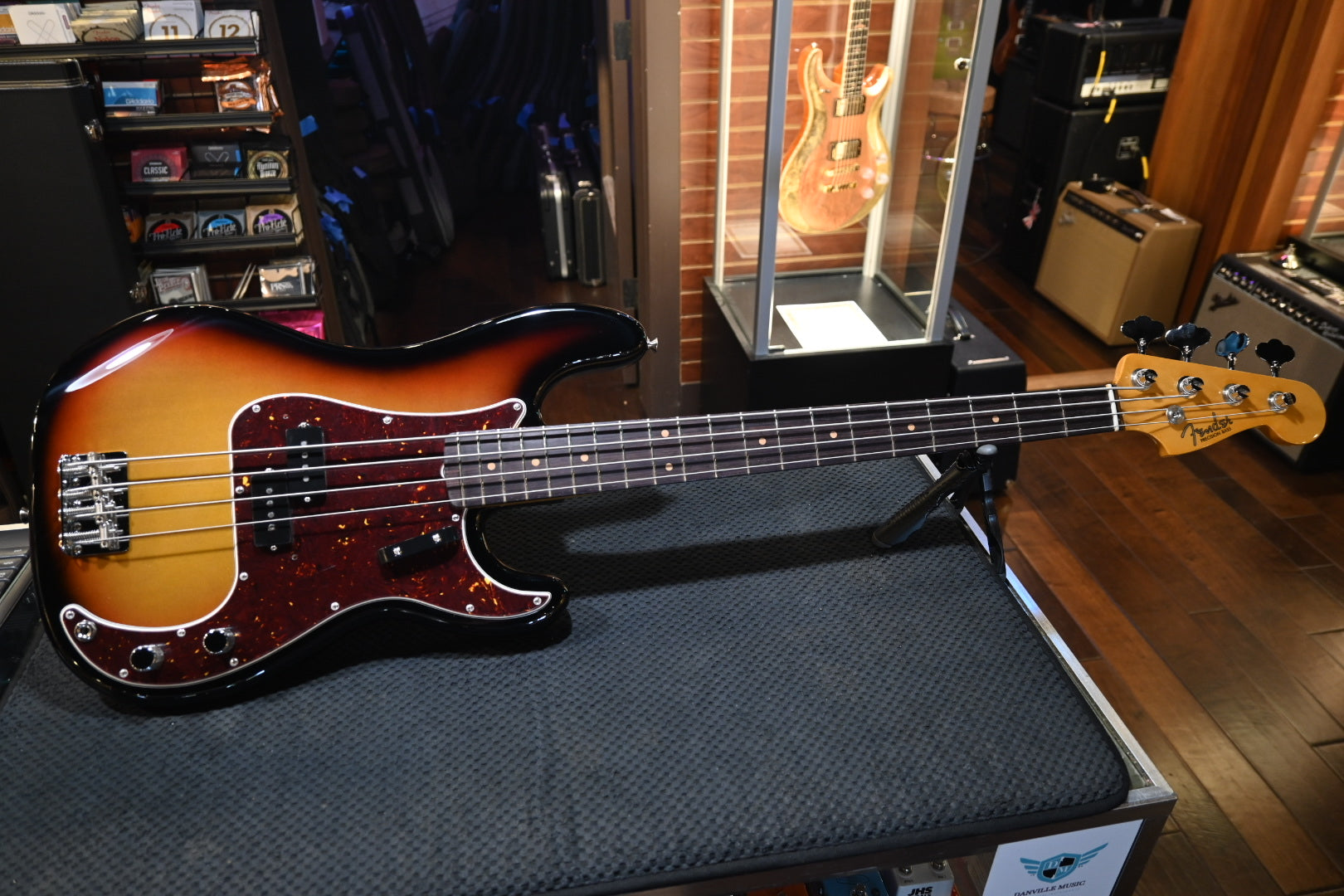The image is a detailed photograph of the inside of a guitar shop. The focal point is an electric guitar resting on a padded cloth shelf that spans from the bottom left to bottom right of the frame. The guitar's design is striking, featuring a vibrant mix of yellow, black, and red with shiny sparkles, includes an orange stripe with black trim and a marble brown section. Its silver steel strings stretch across to the headstock, which is oriented left with four black tuning pegs.

In the background, a lit-up glass case prominently displays another guitar, which is a combination of yellow, tan, and white, glowing under the lights. Behind this, there are several music cases on the floor, each marked with small blue tags or tape. Adjacent to the main guitar, a display shelf holds rows of music CDs, with visible labels numbered 11 and 12. The top right of the image reveals a window and various boxes for sound equipment or other musical accessories.